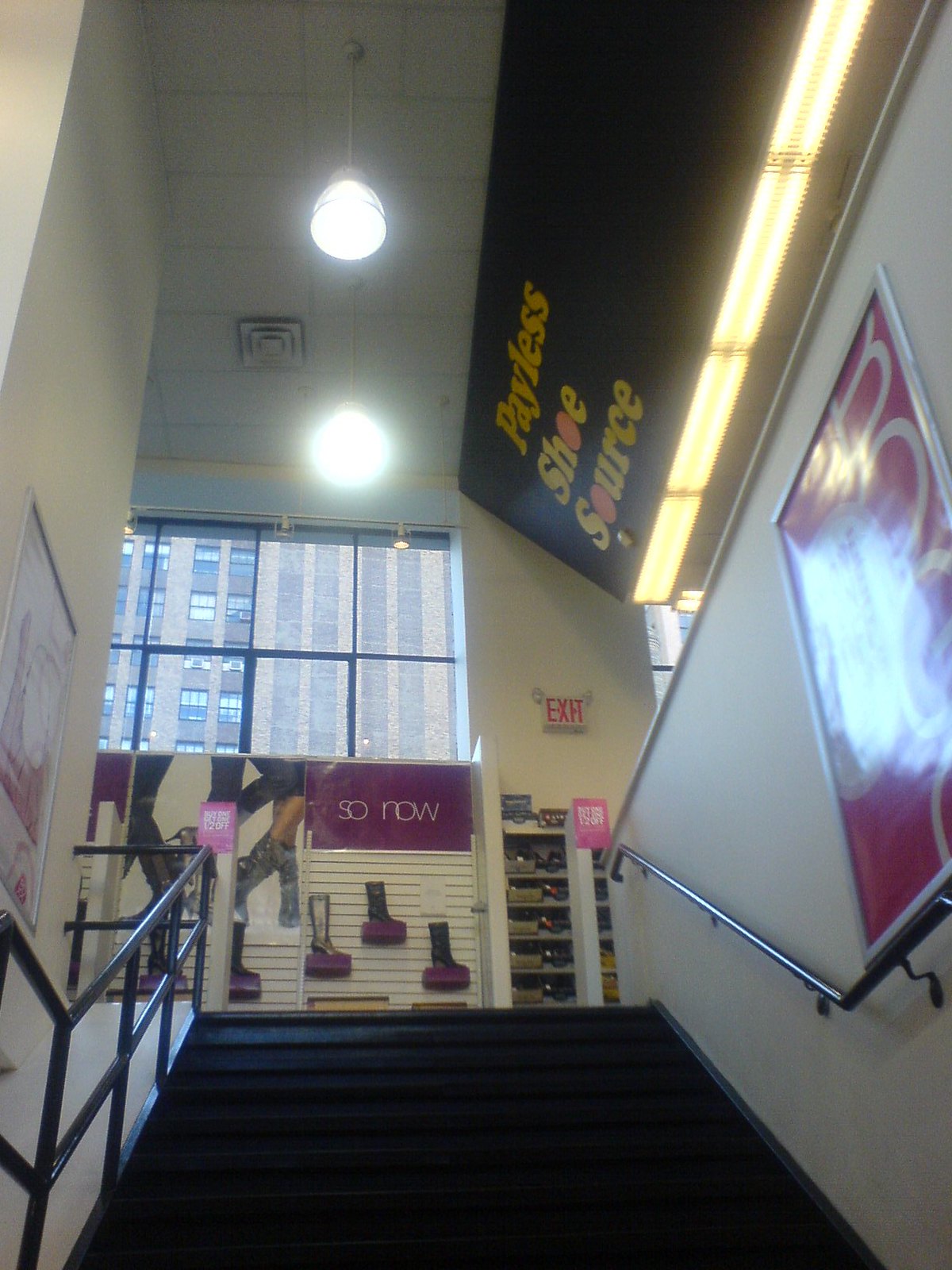This photograph captures the entrance of a Payless ShoeSource store, which appears to be located on an upper floor, accessible via a black staircase. The staircase comprises at least a dozen steps with a black railing on the left side for safety and a beige wall on the right side, equipped with a handrail. A prominent pink poster featuring the "BOGO" (Buy One, Get One) promotion in white letters is affixed to the wall. Additional pink promotional signs are visible along the stairs. 

As one ascends the stairs, a display for boots becomes visible, featuring a burgundy banner with an image of people wearing various boot styles. The display includes at least five boots in different colors, including silver and brown. Adjacent to this, shelves filled with shoes line the right side. An exit sign is mounted near the ceiling, positioned above these shelves.

Above the entrance, a black banner with yellow lettering spells out "Payless ShoeSource," and the ceiling is fitted with white tiles and illuminated by two small lamps, casting a glow over the scene. The presence of large windows reveals an urban setting with numerous high-rise buildings in the background, suggesting a city environment.